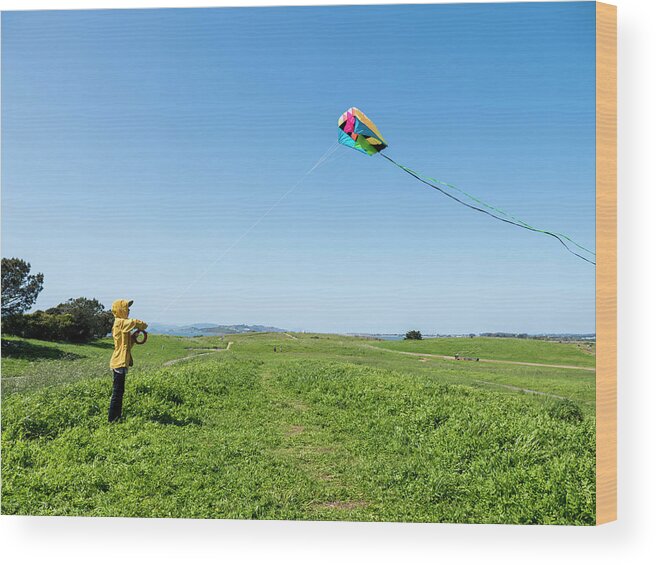The outdoor scene captures a child, who could be either a boy or a girl, joyfully flying a colorful box-style kite in a vast, slightly hilly field of green grass. The child is dressed in a bright yellow long-sleeve shirt, a yellow hat, and dark pants, firmly gripping a reel of line. The vibrant kite, consisting of pink, blue, orange, and green sections, trails a lengthy, dual-colored tail with one stream of green and one of blue. The sky above is an expansive, clear gradient of bright blue transitioning to a lighter shade near the horizon, with no clouds in sight. Surrounding the child, a few green trees and a small crop of bushes add to the picturesque landscape. In the distance, there are hills or mountains, possibly with a body of water nearby. Despite the slight variations in description, the essence of the image is of a serene, sunny day with a child enjoying kite flying against a stunning natural backdrop.